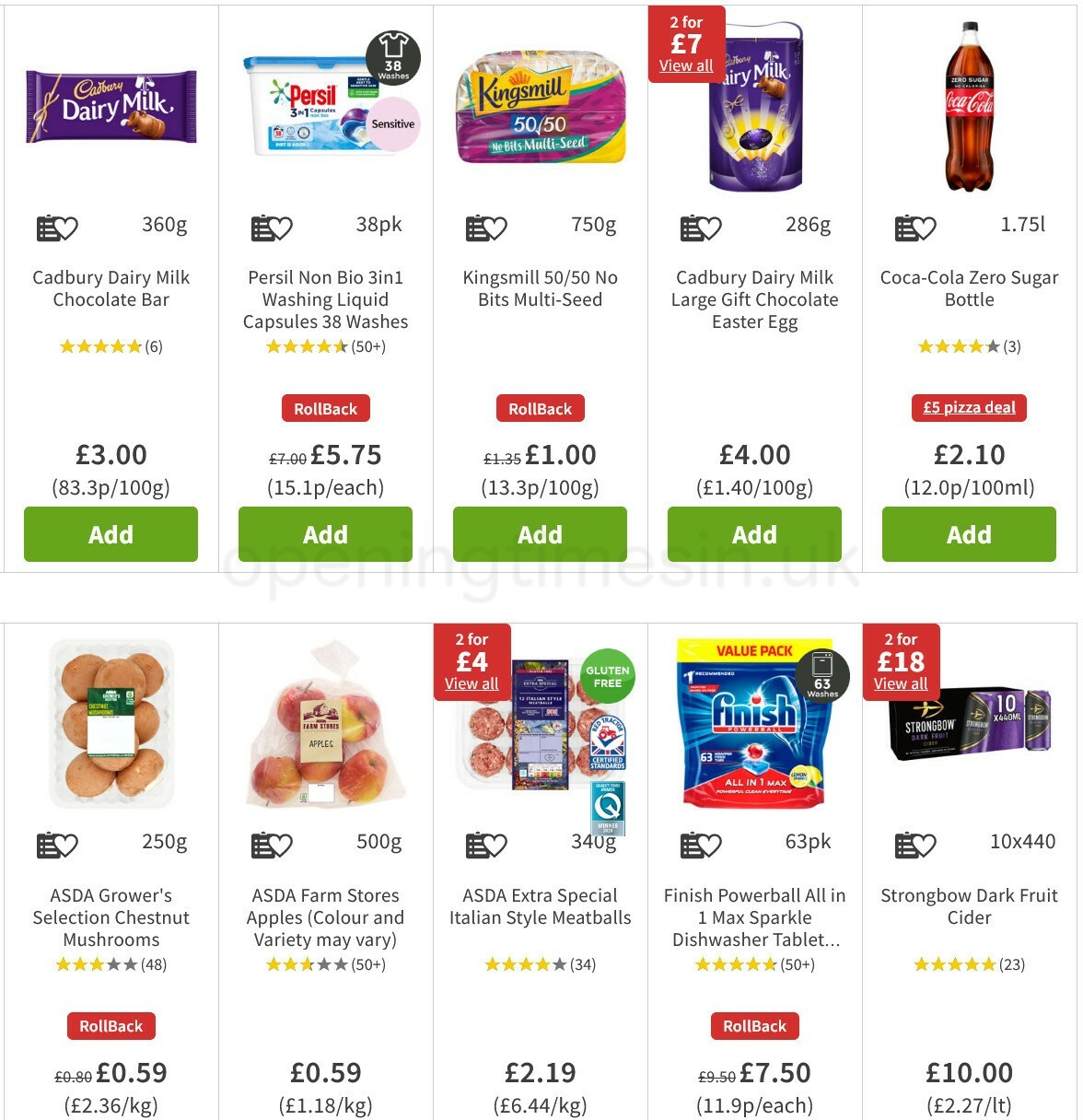This detailed image displays a UK-based online grocery store, featuring prices in pounds. Starting from the left, there's a Cadbury Dairy Milk Chocolate Bar weighing 360 grams, highly rated with an average of four to five stars and costing £3.00, which equates to 83.3 pence per 100 grams. Next to it, there's Persil Non-Bio 3-in-1 Washing Liquid Capsules, suitable for 38 washes, accompanied by an impressive rating of 4.5 out of 5 stars. These are currently on sale with rollback pricing, available for £5.75, breaking down to approximately 15.1 pence per capsule. Further along, we see Kingsmill 50/50 No-Bits Multiseed bread, which seems to be a type of multi-seed bread with a smooth texture, though the exact details and price are not entirely clear from the given description.